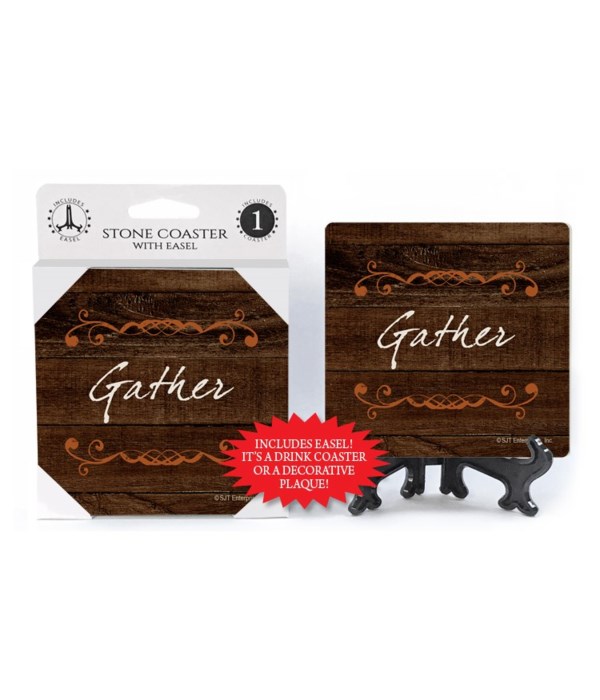The advertisement features a drink coaster with an easel set against a white background. The product packaging prominently displays the text "Stone Coaster with Easel" and highlights that it includes one coaster and one easel. The coaster itself boasts a rich, dark brown, wooden-like texture with an orange etching that resembles a floral vine. Below this design, the word "gather" is written in striking white letters. To the left, the coaster is shown inside its packaging, a white cardboard with clean, bold black lettering, including a number one in a black circle. To the right, the coaster is presented on a black easel, clearly showing its dual function as either a drink coaster or a decorative plaque. Additionally, a red dialog box situated between the two images emphasizes the inclusion of the easel and the versatility of the coaster with exclamatory notes, stating, "Includes easel! Drink coaster or decorative plaque!"